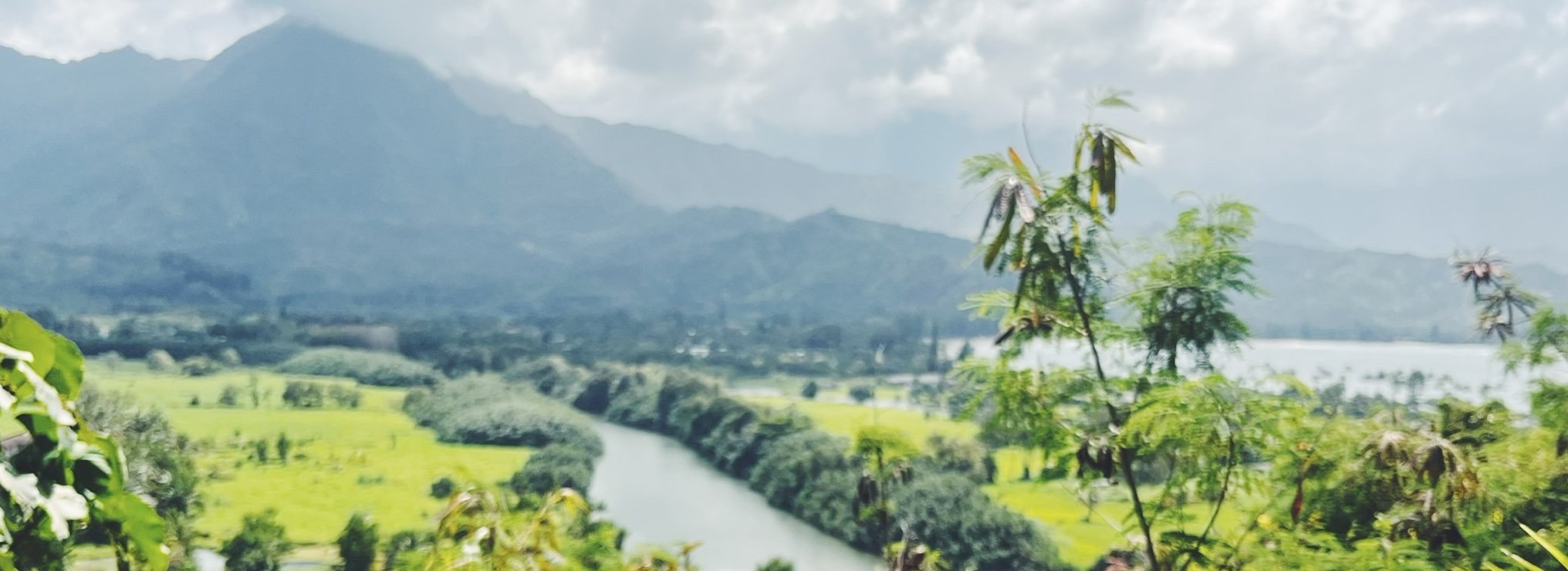This image captures a serene, forested landscape taken during the daytime. The sky is overcast with thick, white clouds, completely obscuring any blue sky. In the background, a range of large mountains extends from the left to the right of the image, gradually fading into a foggy distance. In the middle of the picture, there is a river or canal flanked by bushes, flowing down the valley. Surrounding the waterway, the ground is lush with grass and green plants, creating the appearance of a vibrant, almost tropical forest floor. On the right side of the image, the water continues, suggesting a connection to a larger body of water like an ocean or river. The foreground features zoomed-in views of green plants with leaves, adding to the rich, natural tapestry of the scene. There are no people or text visible in the picture, emphasizing the untouched beauty of the landscape.